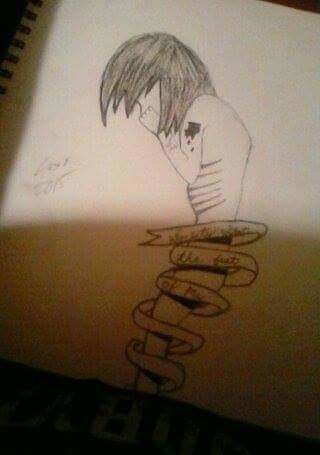A sheet of plain white printer paper rests within a notebook, clearly bound with black metal spirals on its left side. The notebook appears to be placed on a dark blue sheet, adorned with light blue text. The image on the paper depicts a peculiar figure: a man whose body transitions into a stick-like form below his waist. He gazes downward with an expression that suggests sadness. Wrapped around his legs, waist, and bottom is a banner that features unreadable text, with fragments decipherable as starting with a "W," an "S," and possibly a "B," alongside the phrase "the something of me."